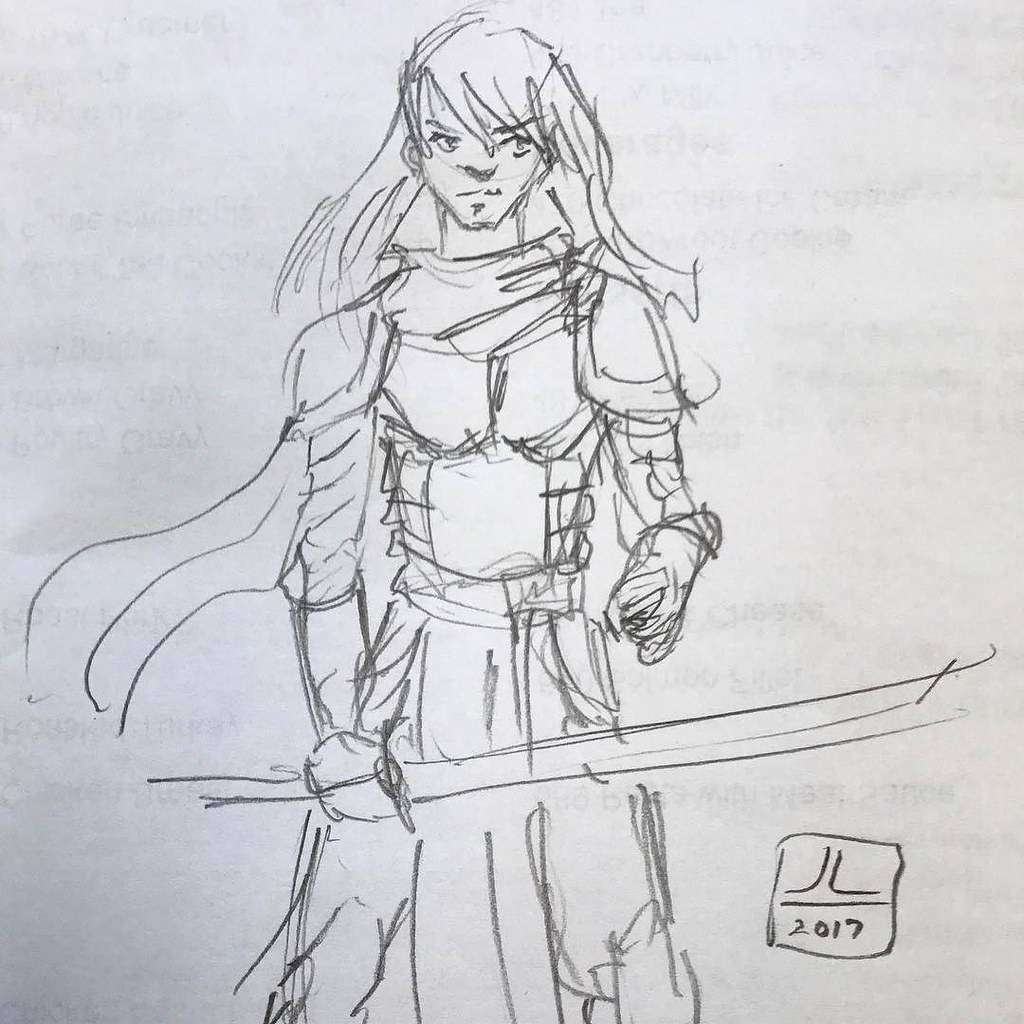A detailed pencil sketch of a male samurai or warrior, meticulously drawn on a piece of white paper. The faint impression of writing from the other side of the paper subtly emerges through the sketch, indicating that the artist chose to doodle on the blank side of an already-used sheet. The warrior is depicted with a formidable breastplate and shoulder armor, accompanied by a flowing cape cascading from his back. His gloved right hand firmly grasps a horizontally positioned sword across his body. The attire includes long, billowing pants that could be mistaken for a skirt at a glance. The artist has marked their creation with a signature: "JL / 2017," enclosed in a small box at the corner of the drawing.